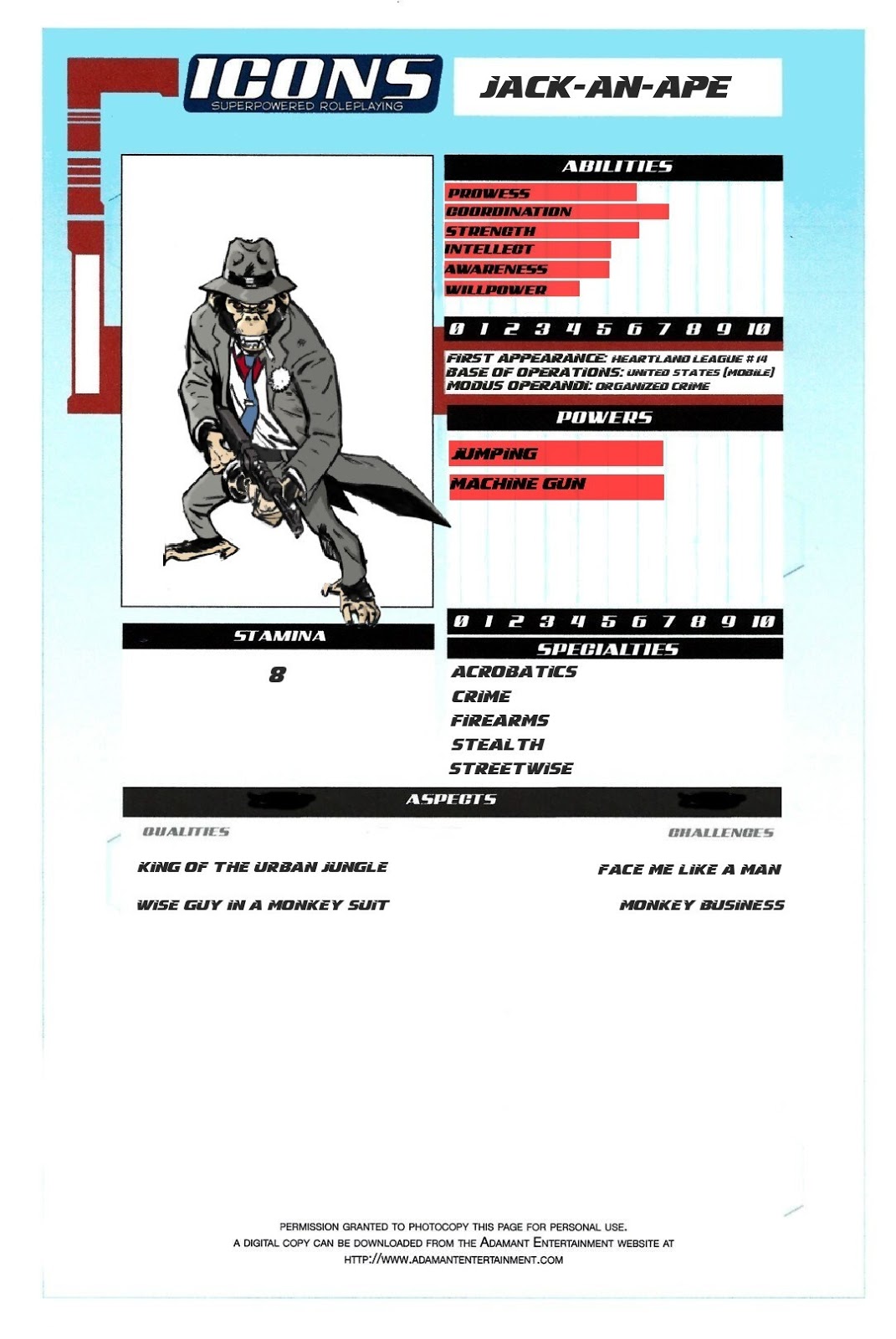The image features a stylized illustration of an ape character dressed in a gray suit, top hat, and blue tie, wielding a machine gun. The background consists of a white, red, and light blue color scheme, with various text elements and statistical information indicating this is likely a depiction from a video game or comic book. At the top, the word "Icons" is prominently displayed in white letters against a blue background, followed by "Jack-N-Ape" in black letters on a white background. 

On the left side of the image, the text "Stamina" is located beneath the illustration of the ape. On the right side, a chart labeled "Abilities" lists various attributes including prowess, coordination, strength, intelligence, awareness, and willpower, depicted with progress bars in red and black. Below this are numerical values ranging from 0 to 10 in white letters on a black background.

Further down, the text "First Appearance" mentions "Heartland League," and "Base of Operations" specifies "United States." This information is followed by a section labeled "Powers," listing special abilities such as "Jumping" and "Machine Gun." Additionally, there is a "Specialties" section detailing traits like acrobatics, crime, firearms, stealth, and streetwise.

The "Aspects" section includes phrases like "King of the Urban Jungle," "Face Me Like a Man," "Monkey Business," and "Wise Guy in a Monkey Suit," adding flavor to the character's persona. The overall design and layout, combined with the unique visual elements, imply this image is part of a larger entertainment medium, potentially a video game or comic book series.